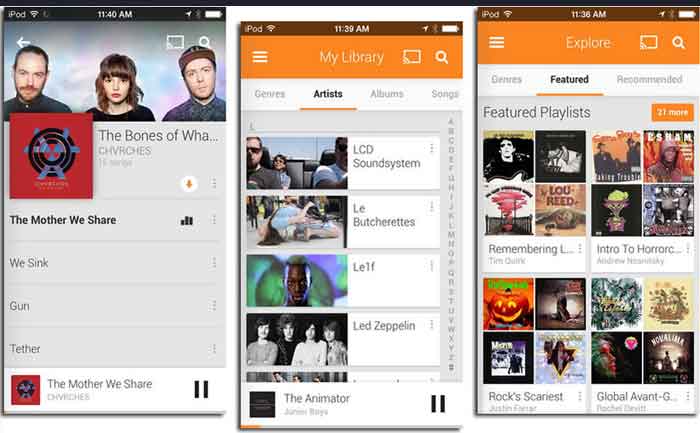The image is a collage of three different screenshots from an old iPod Touch, each showcasing various functionalities and screens of the device’s music library interface.

1. **First Screenshot - Album View**
   - The first screenshot displays a list of songs from an album titled "The Bones of What," although the full title is cut off. The artist is CHVRCHES, stylized with a "V" for the "U." The songs visible from this album are:
      - "The Mother We Share" (bolded to indicate it is currently playing)
      - "We Sink"
      - "Gun"
      - "Tether"
   - At the bottom of this screen, there is an option to pause the currently playing song, "The Mother We Share." The top of the screen depicts a banner image of the band members: two Caucasian males flanking a Caucasian female.

2. **Second Screenshot - My Library**
   - The second screenshot showcases the “My Library” section, with the "Artists" option highlighted. The unselected options are “Genres,” “Albums,” and “Songs.”
   - Listed artists include:
      - LCD Soundsystem
      - Le Butcherettes
      - Leaf
      - Led Zeppelin
   - The song currently playing at the bottom of this screen is "The Animator," though the artist's name is not visible.

3. **Third Screenshot - Explore**
   - The final screenshot displays the "Explore" section, with "Featured" highlighted among the categories “Genres,” “Featured,” and “Recommended.”
   - Under "Featured," it lists several playlists with album covers, but the text fields are not large enough to display the full names of some playlists. Visible names include:
      - "Remembering…" (possibly an incomplete title)
      - "Intro to Horrorcore"
      - "Rock’s Scariest"
      - "Global Avant-Garde" (though the word "Avant-Garde" is cut off)
   
Combined, these images offer a nostalgic glimpse into the music navigation experience on an old iPod Touch, highlighting specific albums, artists, and playlists within the device's library.